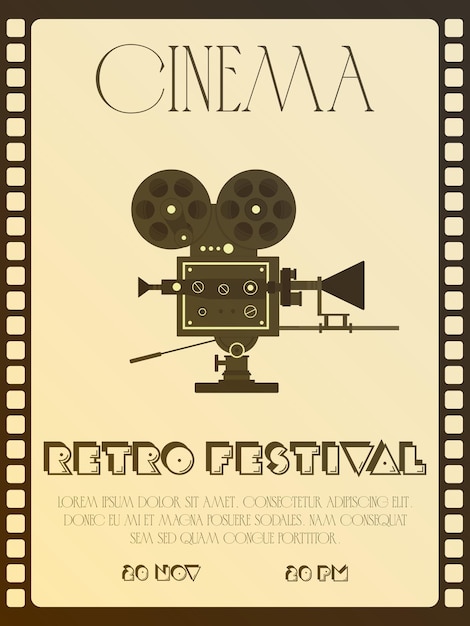The image is an old-fashioned cinema festival advertisement poster designed to resemble a vintage film reel. The poster features a frame with empty film reel sprocket holes running down the left and right sides on a light yellow or tan background. At the top, in large serif-style black text, it says "Cinema." Below this, there is an illustration of an old-fashioned camera or projector, depicted in black and white or a dark greenish color with two prominent reels. Beneath this image, in large white bubble letters against a dark brown background, it reads "Retro Festival." Further down, the poster provides event details in a light gray font that appears to be in Latin placeholder text, and bold bubble letters specifying the date and time: "20 NOV" at 20 PM.